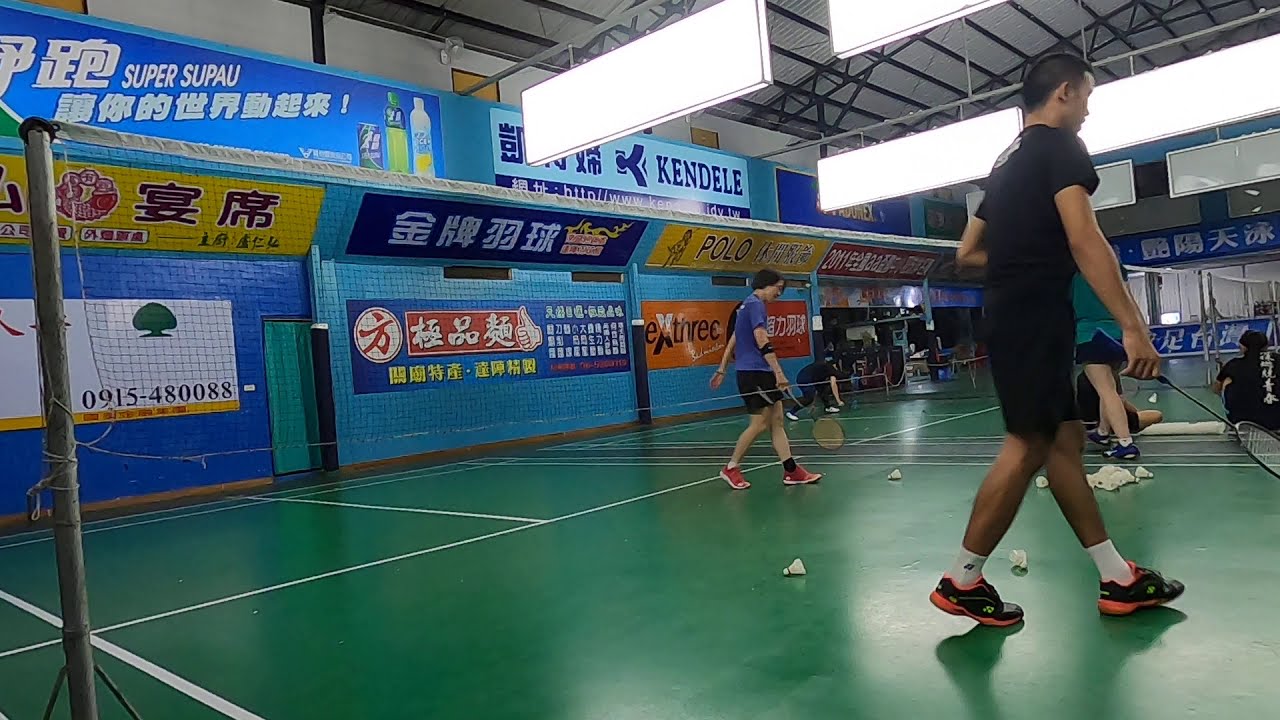The image depicts a bustling indoor badminton court with a green surface marked by white lines. Dominating the center is a regulation badminton net, extending from left to right, held up by silver poles. In the background, a blue-tiled wall adorned with a multitude of banners in various foreign languages adds a vibrant touch, with one prominent white banner bearing the number 0915-480088. Near the top, a light blue banner displays the letters "KENDLE." 

A group of people, around five or six, are walking towards the right side of the image. At the forefront, a man clad in a black shirt and shorts, black shoes with orange soles, and white socks strides confidently. Directly behind him, another individual in a blue shirt, black shorts, and red shoes holds a badminton racket, its head pointed downwards. Scattered on the court are several badminton shuttlecocks.

The ceiling above features an arrangement of bright, rectangular light fixtures with red linings, suspended from a network of black girders supporting a white roof. In the distance, large windows provide a glimpse into another section of the facility, suggesting a spacious, well-lit recreational venue teeming with activity.